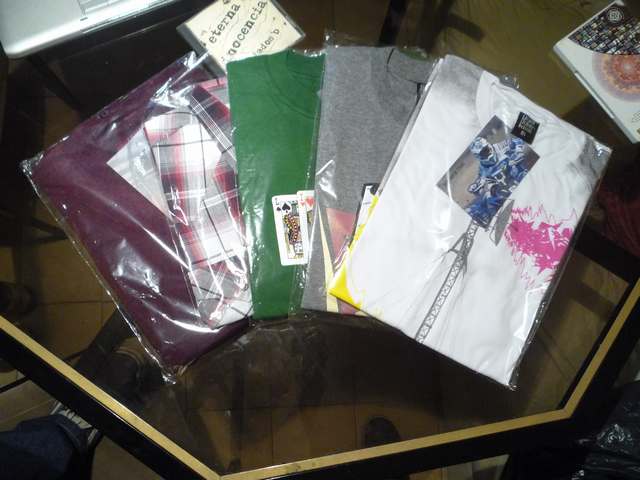This image features a hexagonal glass table with a gold or bronze-colored frame, showcasing five neatly folded, plastic-wrapped t-shirts. Positioned on the table from right to left, the first shirt is white with a gray and pink design, partially obscuring a small photograph of a person wearing a bicycle helmet. Next is a gray t-shirt with unknown graphics, followed by a green t-shirt displaying unconventional playing cards with letters 'L' and 'I'. Situated to the left of these is a red, gray, and white checkered shirt, and lastly, a maroon-colored shirt. Visible beneath the tabletop are a person's dark pant leg and white sneaker, with an assortment of indistinguishable objects scattered across the table, including a sticky note and a computer-related item.